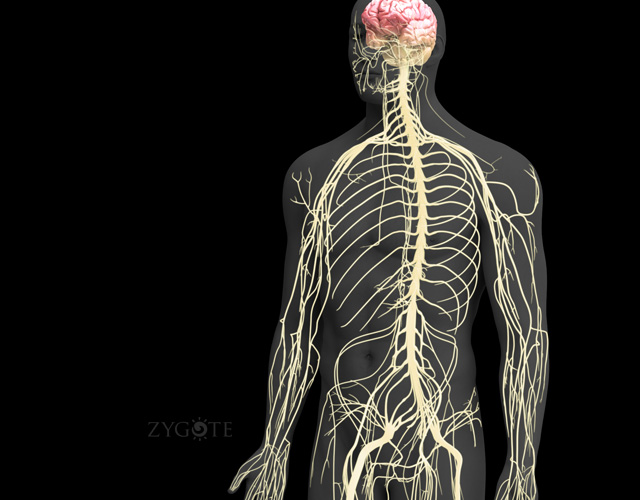The image depicts an artistic, abstract representation of the human nervous system set against a completely black background with no variations. The piece is credited to an artist named Zygote, as indicated by a watermark on the image. The figure, resembling a man's body, appears as a silhouette, with the internal structure portrayed in a fluid, almost x-ray-like manner. The primary focus is the intricate network of nerves depicted in a light yellowish-green color, extending from the head down to just below the hips. Notably, the brain stands out with a bright pink hue, although the very top part of the head and brain is slightly cut off. Elements like the belly button and the spine are visible, adding fine details to the otherwise shadowy figure. The image blends scientific recreation with artistic expression, offering a unique, visually captivating depiction of the human nervous system.